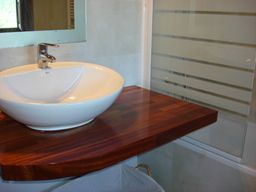A compact photograph showcases a sleek bathroom sink basin positioned elegantly in the corner. The basin, crafted from shiny white porcelain and designed in a chic bowl shape, rests on a polished dark reddish-brown natural wood surface. The wood surface, finished impeccably, exhibits distinctive grain patterns and stands above an open space where a white laundry basket or rubbish bin resides. The sink is highlighted by a small, centrally-placed chrome faucet that gleams under the light. Above the sink, a small cabinet or mirror with a prominent aluminium-colored border reflects the surroundings. The mirror is mounted on a wall adorned with white tiles featuring subtle grey accents, adding a touch of sophistication. Adjacent to the sink, a glass shower screen with frosted panels and horizontal clear lines provides a stylish decorative element, hinting at the modern design of the bathroom.